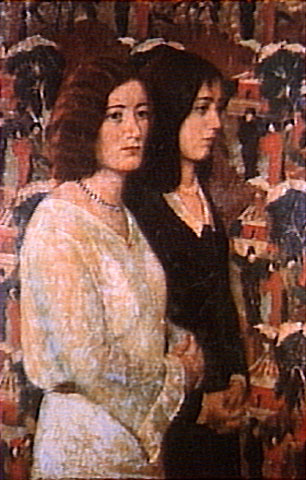This painting, which is astonishingly realistic and almost photo-like, depicts two somber women standing side-by-side. Both women display expressions of sadness and contemplation, their eyes cast downward, and their hands folded in front of their stomachs. The woman on the left, characterized by her dark red, almost brown, curly hair, wears a long, cream-colored dress with slightly ruffled wrists, and a silver necklace around her neck. Her companion on the right has straight black hair, shoulder-length, and is dressed in a black dress with a white collar, also donning a necklace. Both women have pale skin and stand against a blurred background that resembles a wallpaper pattern. This backdrop features small, repeated figures in red and black, resembling people, houses, and trees, contributing to the slightly ambiguous setting that evokes a sense of being in a church or some form of solemn event.